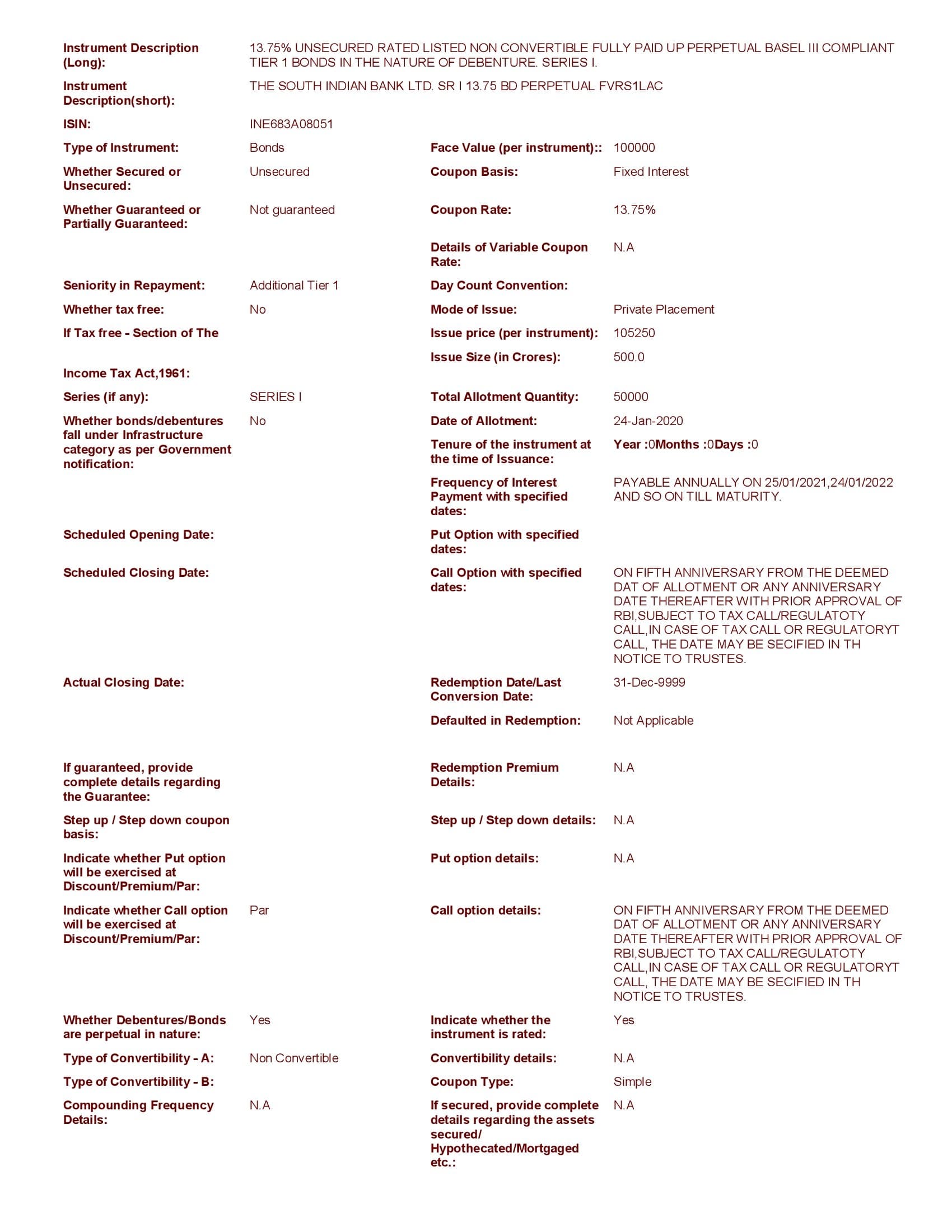**Detailed Caption:**

The image is a densely packed screen capture detailing financial information about bonds. The text is heavily information-laden, with brown bold text on the left side and organized into two distinct columns. The content varies based on the type of financial instrument under discussion.

For example, one section starts with an 'Instrument Description: Long' detailing a 13.75% unsecured bond, rated, listed, non-convertible, and fully-paid up, perpetual, BASE III compliant Tier One bond. This description is classified under the 'Nature of Debenture: Series I'. The short description for the same instrument reads: "The South Indian Bank Limited SR 113.75 BD Perpetual," with a face value of Rs. 1 Lakh and an ISIN number of INE 683A 08051. The instrument type is listed explicitly as bonds with a face value per instrument of $100,000, indicating it is unsecured.

The coupon basis is fixed interest, with additional details about whether the bond is guaranteed or partially guaranteed (it is not guaranteed) and states the coupon rate at 13.75%. Information on variable coupons is unavailable. The second column continues with information related to face value and coupon details.

The document also mentions the closing date and contains copious legal details that explain why the South Indian Bank, issuing the bond, is legally required to disclose this information. The extensive legal language and the volume of detailed information would require approximately five minutes to thoroughly read and comprehend.